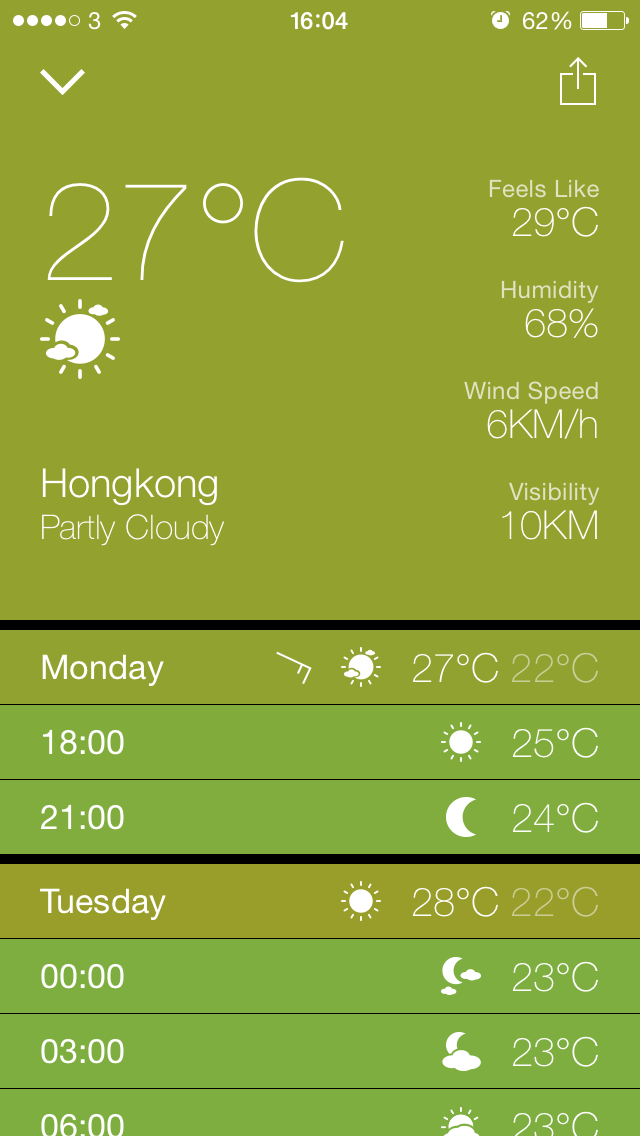The image displays a detailed weather report for Hong Kong against a green background. In the top left, the time reads 16:04, alongside a battery indicator showing 62%. An alarm clock icon is present, along with the current temperature of 27°C, which feels like 29°C. The humidity is at 68%, depicted next to sun and cloud icons, and the wind speed is 6 km/h with a visibility of 10 km. 

Underneath, the information is divided into relevant sections:
- **Current Weather**: Shows partly cloudy conditions with the temperature at 27°C.
- **Daily Forecast**: 
   - **Monday**: The highs and lows are 27°C and 22°C respectively. The forecast for 18:00 shows 25°C with a sunny icon. At 21:00, the temperature is 24°C with a moon icon.
   - **Tuesday**: The rectangles indicating the days are orange, showing a high of 28°C and low of 22°C. At 00:00, the weather is depicted with a moon and clouds at 23°C, followed by a time of 03:00.

Overall, the image combines various metrics and icons to present a comprehensive weather update for Hong Kong, detailing temperatures, humidity, wind speed, and visibility for specific times of the day.